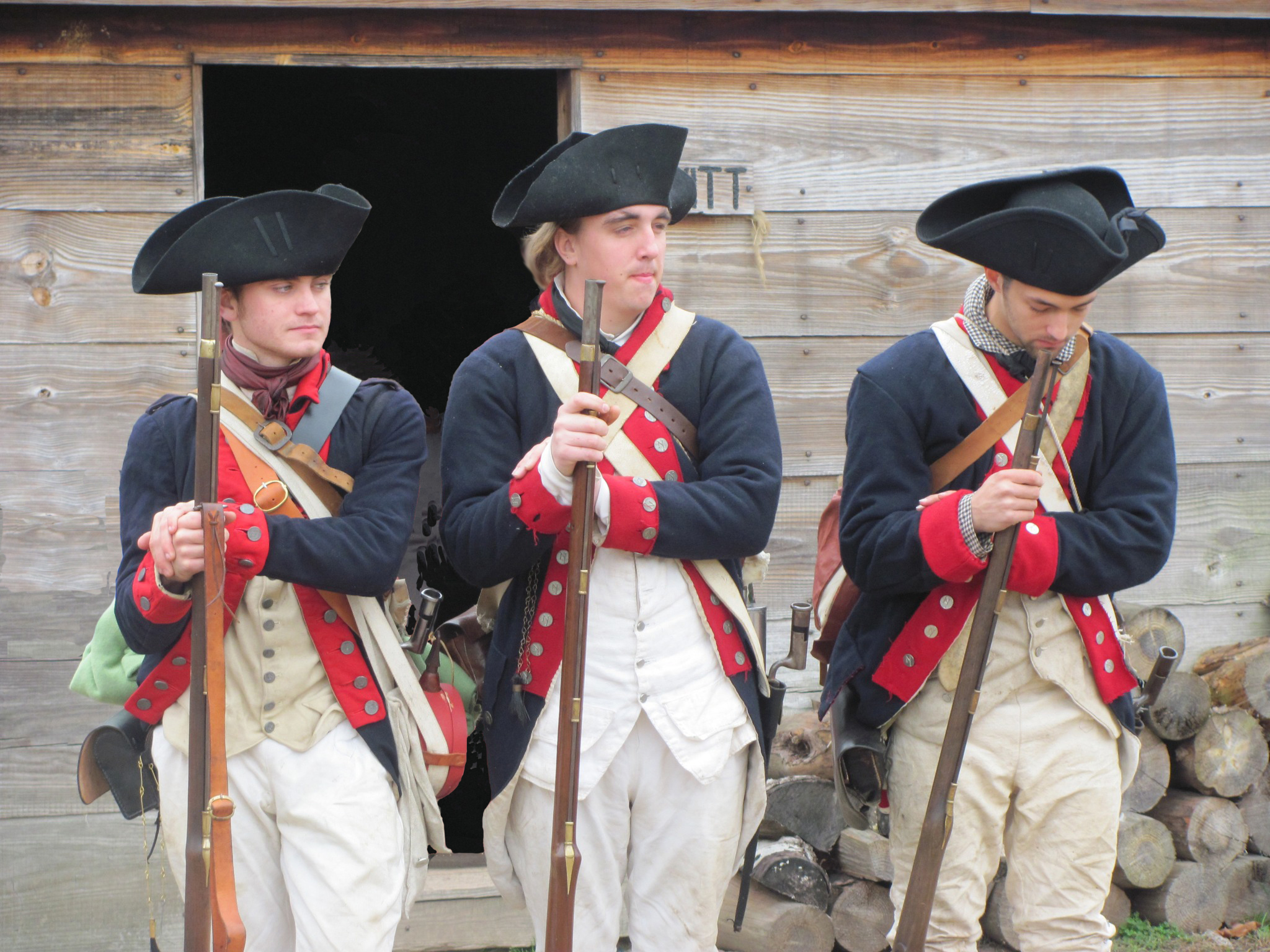This image depicts three young men dressed in colonial marine uniforms from the 1700s, standing in front of a wooden building that resembles a cabin. Each man is holding a rifle upright with his right hand, while his left hand rests on the wrist of his right hand. They are posed side by side, facing slightly to their left, with the man on the right looking downward. Their uniforms consist of black tricorn hats, navy blue jackets with red trim and white buttons, white button-up shirts, and white pants. They wear red belts and crisscrossed white straps across their bodies, adorned with various small items such as pocketbooks and canteens.

Behind them, a partially open door reveals a dark interior, and on the right side of the door, a sign ending with the letters "TT" is visible. A pile of chopped logs is situated behind the men on the right, and the wooden structure of the building features a gradient from grayish tones at the bottom to more brown hues at the top. The overall scene gives an authentic historical feel, possibly capturing the essence of a reenactment or cosplay event.